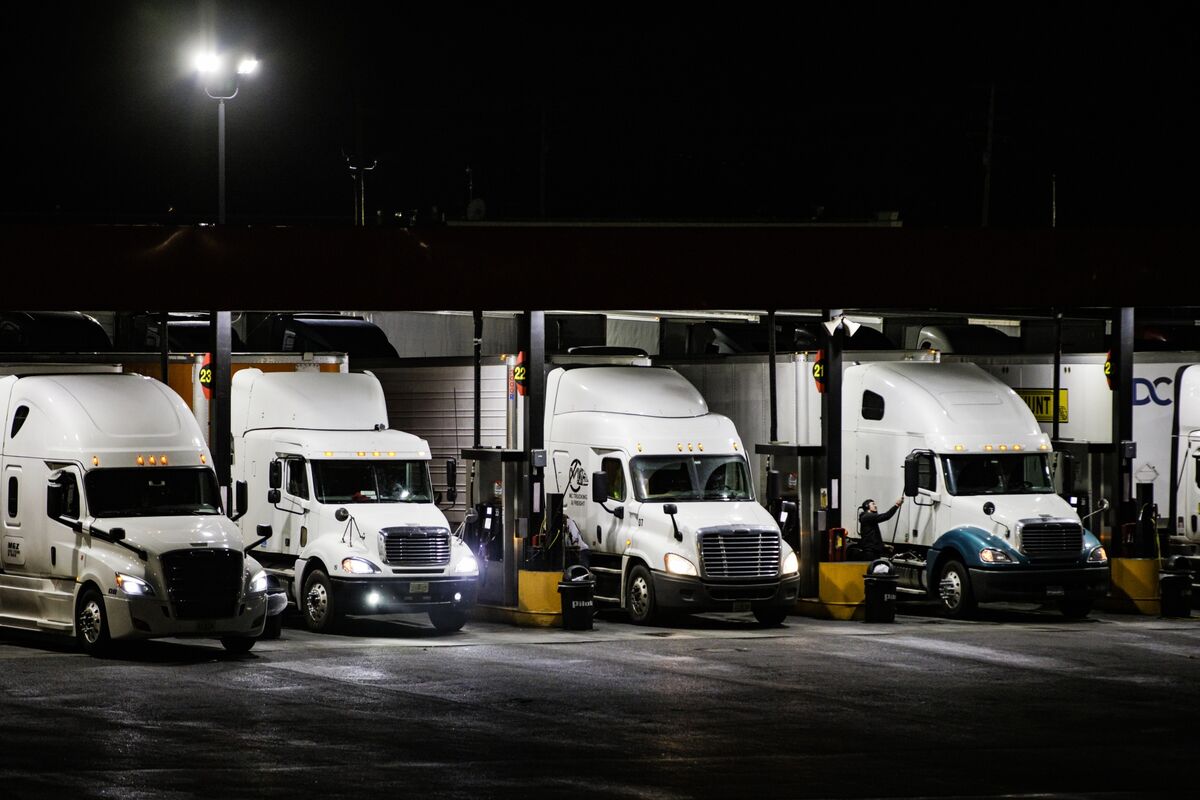This nighttime image captures a scene featuring five large white transport trucks stationed at what appears to be a truck garage or a factory loading area. Each truck is parked in its respective numbered stall, with visible stall numbers 20 through 23. The trucks, the type commonly seen on highways with trailers hitched, have their headlights on, illuminating the area along with bright lampposts scattered around. One corner of the image depicts a man wearing a dark hoodie and headphones, appearing to engage in maintenance or cleaning activities near the trucks. The tranquil nighttime setting is contrasted by the bustling activity around the vehicles, painting a vivid picture of a still, industrious night.